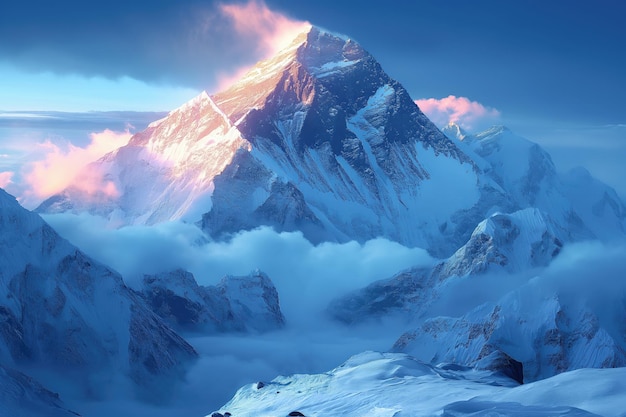The image captures a majestic, snow-covered mountain peak illuminated by the warm hues of a sunrise or sunset. This towering mountain, possibly resembling Mount Everest, rises high above a sea of heavy, billowing clouds that envelop its base and midsection. The left side of the mountain glows with a striking blend of pink, orange, and yellow light, creating a dramatic contrast with the cool blue and white tones that dominate the right side and bottom of the image. Craggy, snow-covered rocks are visible in the foreground, adding to the rugged and imposing nature of this formidable peak. The sky above is filled with gray clouds, but a break at the horizon allows the brilliant sunlight to cast a radiant, almost ethereal glow on the mountain, highlighting its grandeur and perilous beauty.